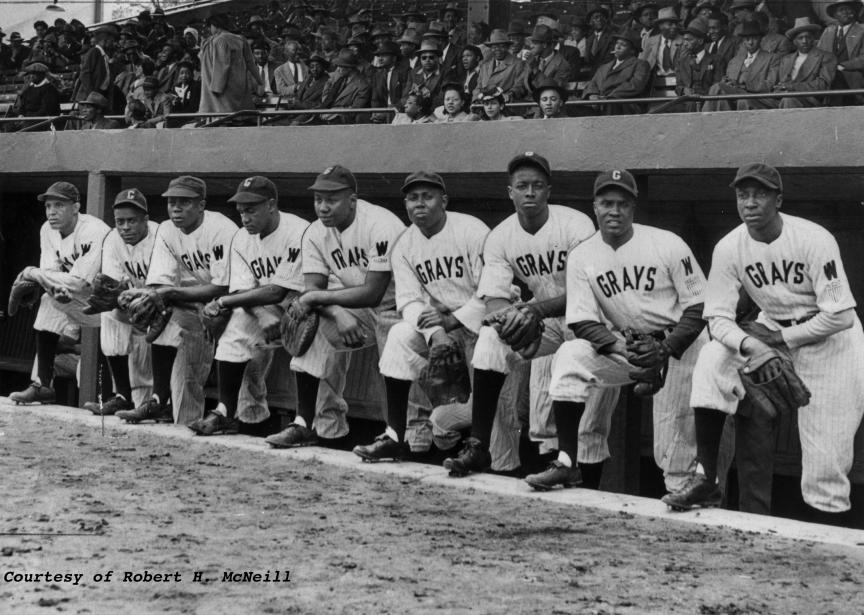This black-and-white photograph, courtesy of Robert H. McNeil, captures a historic moment of a black baseball team, presumably from many years ago. The image features nine players in their dugout, each with one foot on the field and the other inside the dugout, resting their hands on their knees which are positioned outside the dugout. All players are adorned in white uniforms emblazoned with "Grays" in black lettering across their chests. They wear black hats, some marked with a C and others with a G in white. Their uniform pants are white with pinstripes, rolled up above knee-length black socks, and black cleats. Each player holds a baseball glove and poses with an air of poised readiness, arms crossed over their elevated knees. Behind them, the top third of the image reveals a crowd primarily composed of African-American men, dressed in suits and top hats, attentively watching the scene. The rich details of the photograph, including the brown dirt of the field, add texture to this evocative snapshot of a significant era in baseball history.